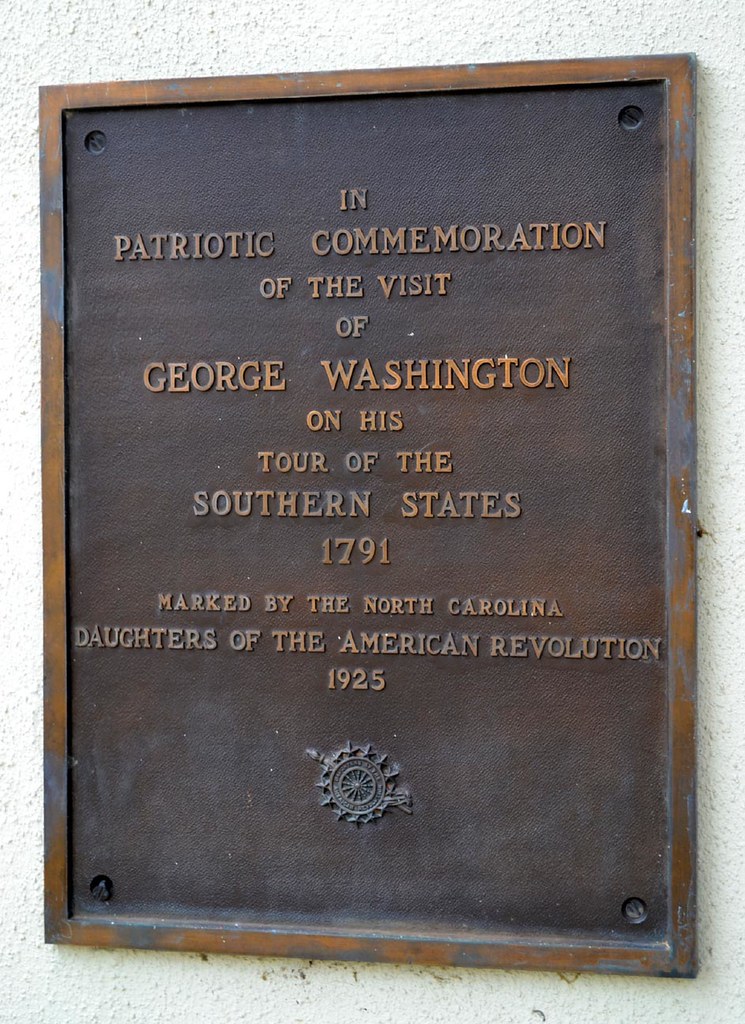This close-up photograph depicts a bronze plaque screwed onto a white concrete wall. The plaque, which shows signs of age with gray discolorations amidst its dark brown, tan, and bronze hues, is secured by four large black bolts, one at each corner. The text on the plaque, in raised lighter copper letters, reads: "In patriotic commemoration of the visit of George Washington on his tour of the southern states, 1791, marked by the North Carolina Daughters of the American Revolution, 1925." Below the text, there is an embossed image that appears to be a wheel with spokes or stars surrounding it and a spear-like object running diagonally from the bottom right to the top left, though it is difficult to make out the details. This plaque is likely affixed to a building or monument honoring George Washington's historical visit.